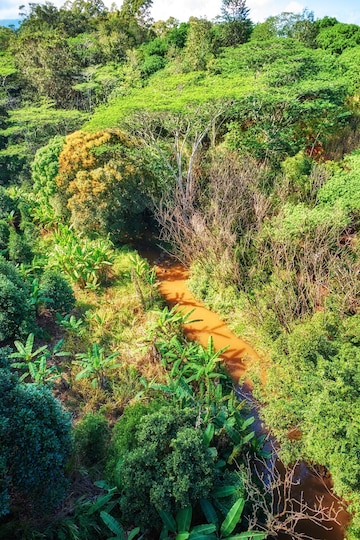The photograph captures a vibrant and lush tropical jungle setting, teeming with a diverse array of dense, green vegetation. Central to the image is a river with an orange, rust-colored hue, likely a result of recent rains causing muddy runoff. The river meanders through the landscape, initially visible but gradually obscured by the thick canopy of towering palm trees, banana trees, and various other tree species. The foliage showcases a rich spectrum of greens interspersed with yellow and orange tints, while the forest is dotted with numerous twigs and branches. This scene unfolds under a bright blue sky sprinkled with clouds, highlighting the natural beauty of a jungle on a sunny day. There are no people or animals present, emphasizing the untouched and serene quality of this outdoor haven.